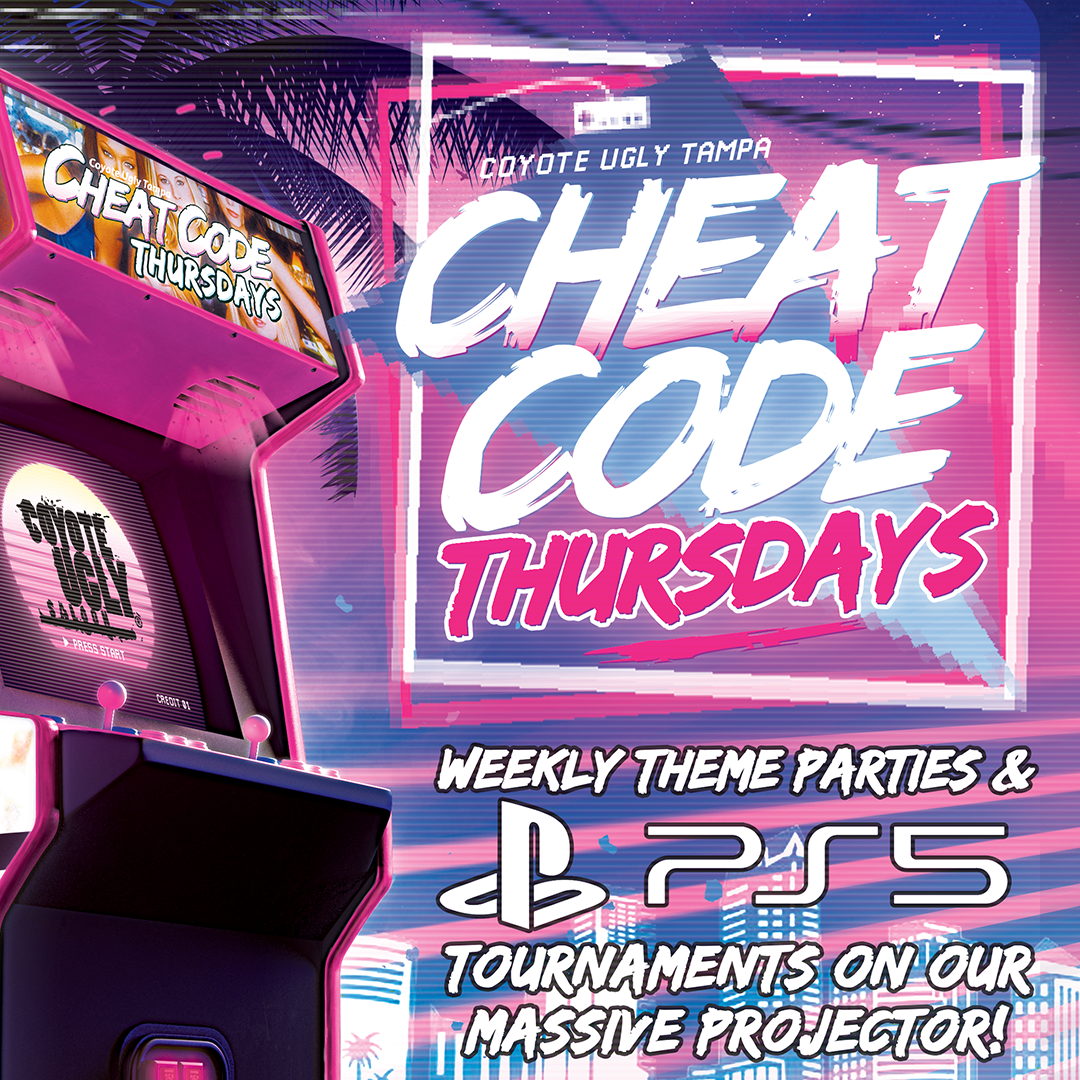The image is an advertisement for "Coyote Ugly Tampa Cheat Code Thursdays." The vibrant poster features a playful, retro theme with pink and blue striped backgrounds, reminiscent of a glitchy, cotton candy aesthetic. On the right side, a white and pink block of text prominently announces "Coyote Ugly Tampa Cheat Code Thursdays," using white font for "Cheat Code" and pink for "Thursdays." Below this, the text promotes "Weekly Theme Parties" and "PS5 Tournaments on our massive projector," with the PS5 emblem included. To the left, a creatively drawn palm tree sits above an old-fashioned arcade machine. This arcade, designed with pink knobs and a black base, displays "Cheat Code Thursdays" at the top and "Coyote Ugly, Press Start" within a lit-up circular screen. The bottom of the image portrays an outlined urban skyline, further enhancing the whimsical, themed atmosphere of the advertisement.